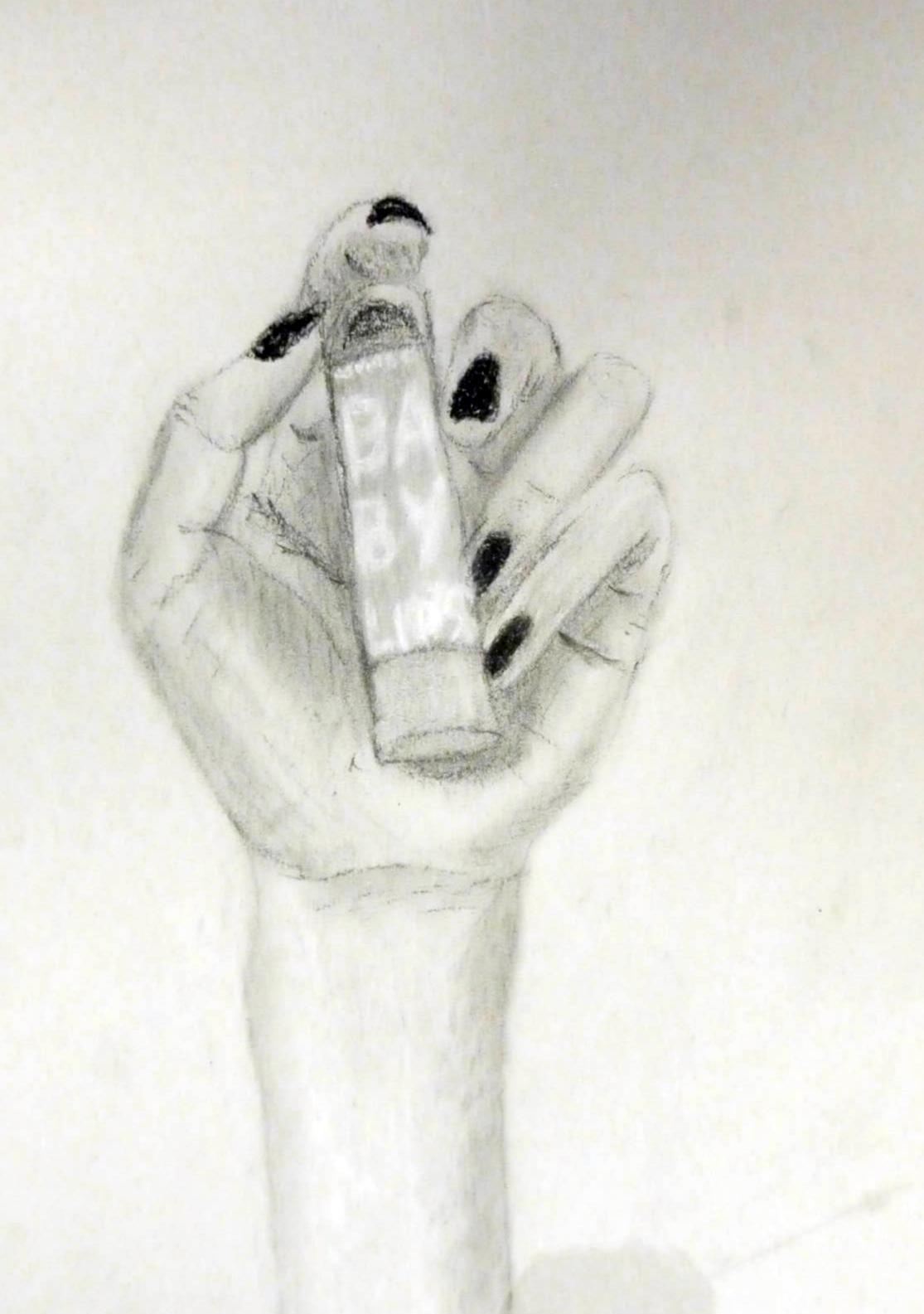This is a soft, charcoal or pencil drawing that appears to be created by a novice artist. The black and white artwork features a white, feminine hand with well-manicured nails painted in a dark color, delicately gripping a tube of lip makeup labeled "baby lips" in white text. The design emphasizes shading to provide a 3D effect, though there are no sharp lines, suggesting an impressionistic style. The hand, shown with some natural curvature and slight distortion, casts a subtle shadow, adding depth. The overall background and composition maintain a gentle, grey-toned softness, enhancing the amateur yet expressive quality of the drawing.